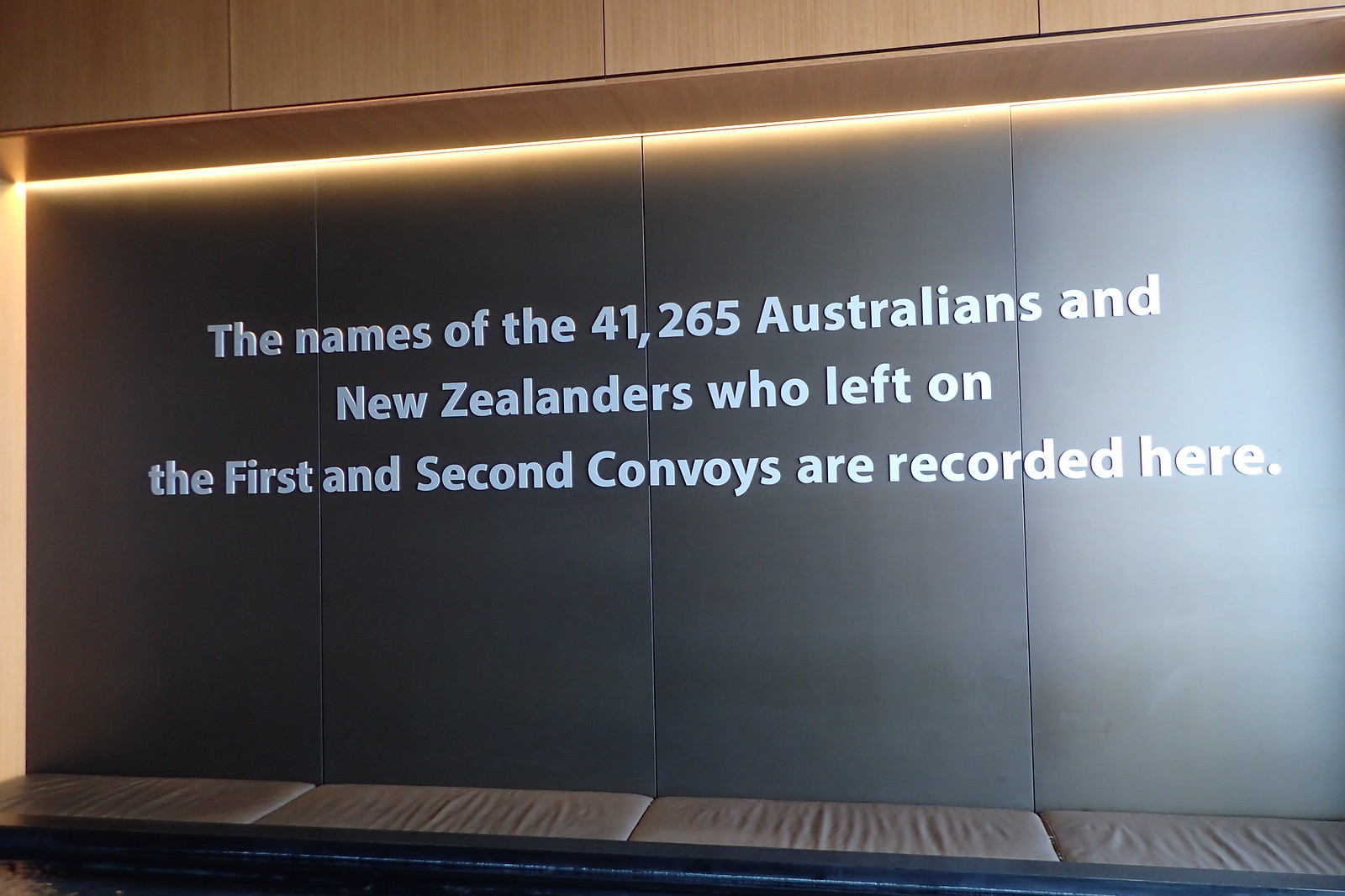The image captures a well-lit indoor setting in a hall or building, featuring a memorial panel. Central to the image is an indented section of wall, dominated by sleek black panels. Positioned in front of these panels is an upholstered bench with rectangular, brown cushions. The black panels display raised white lettering that commemorates the names of the 41,265 Australians and New Zealanders who left on the first and second convoys. Above the memorial text is a wooden-paneled section of wall, prominently illuminated by a backlit fluorescent light, which enhances the clarity of the inscription. Reflections and lighting create a slightly white glare on the right side of the sign, likely from the camera's flash. This descriptive tribute effectively merges the solemnity of the setting with a respectful recognition of history.